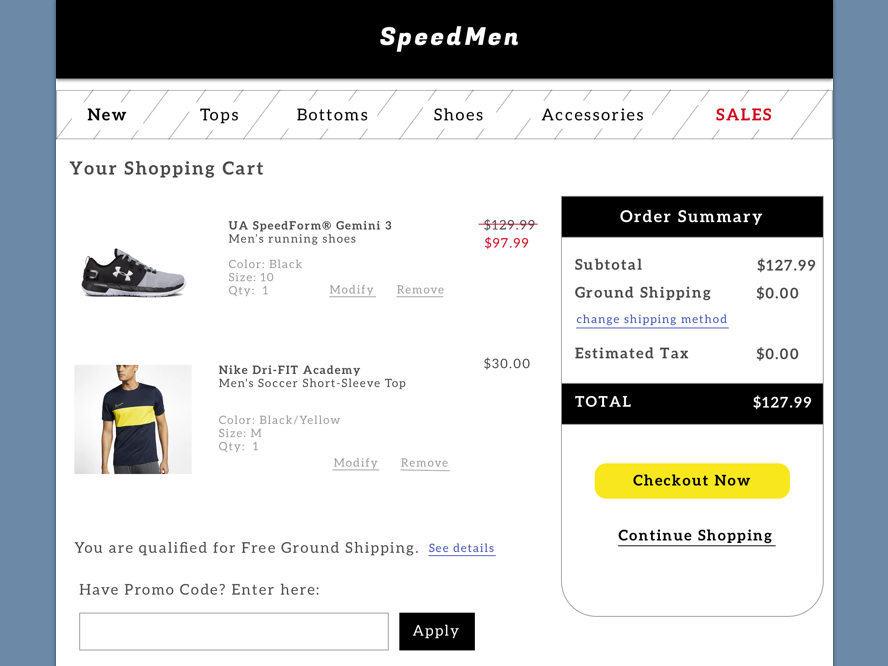The webpage features a sleek black header with the brand name "Speedman" emblazoned in bold white letters at the top center. Adjacent to this, running vertically along each side of the page, are two sidebars.

Directly below the "Speedman" logo, the navigation menu is displayed prominently in black letters, listing categories such as "New," "Tops," "Bottoms," "Shoes," and "Accessories." Highlighted in red letters, the "Sales" category catches the eye for potential bargains. Adjacent to this menu, a shopping cart icon reveals the items selected for purchase.

Inside the shopping cart, an athletic shoe is prominently featured with detailed descriptions: "UA Speed Format Gemini 3 Men's Running Shoe" in black, priced at $97.99, marked in red. The shoe is depicted in black and gray tones.

Below the shoe, a t-shirt is listed: "Nike Dry Fit Academy Men's Soccer Shirt," detailed as a short-sleeve top, priced at $30.00. The shirt is visually described as black with a striking white stripe across the chest.

Beneath these product listings, a notification informs the user about qualifying for free ground shipping with a "See Details" link. There's also a prompt for entering a promotional code, accompanied by a text box and an "Apply" button.

On the right side of the webpage, the "Order Summary" totals the purchase to $127.99. The "Check Out Now" button stands out in yellow, followed by a "Continue Shopping" option in black, underlined for emphasis.